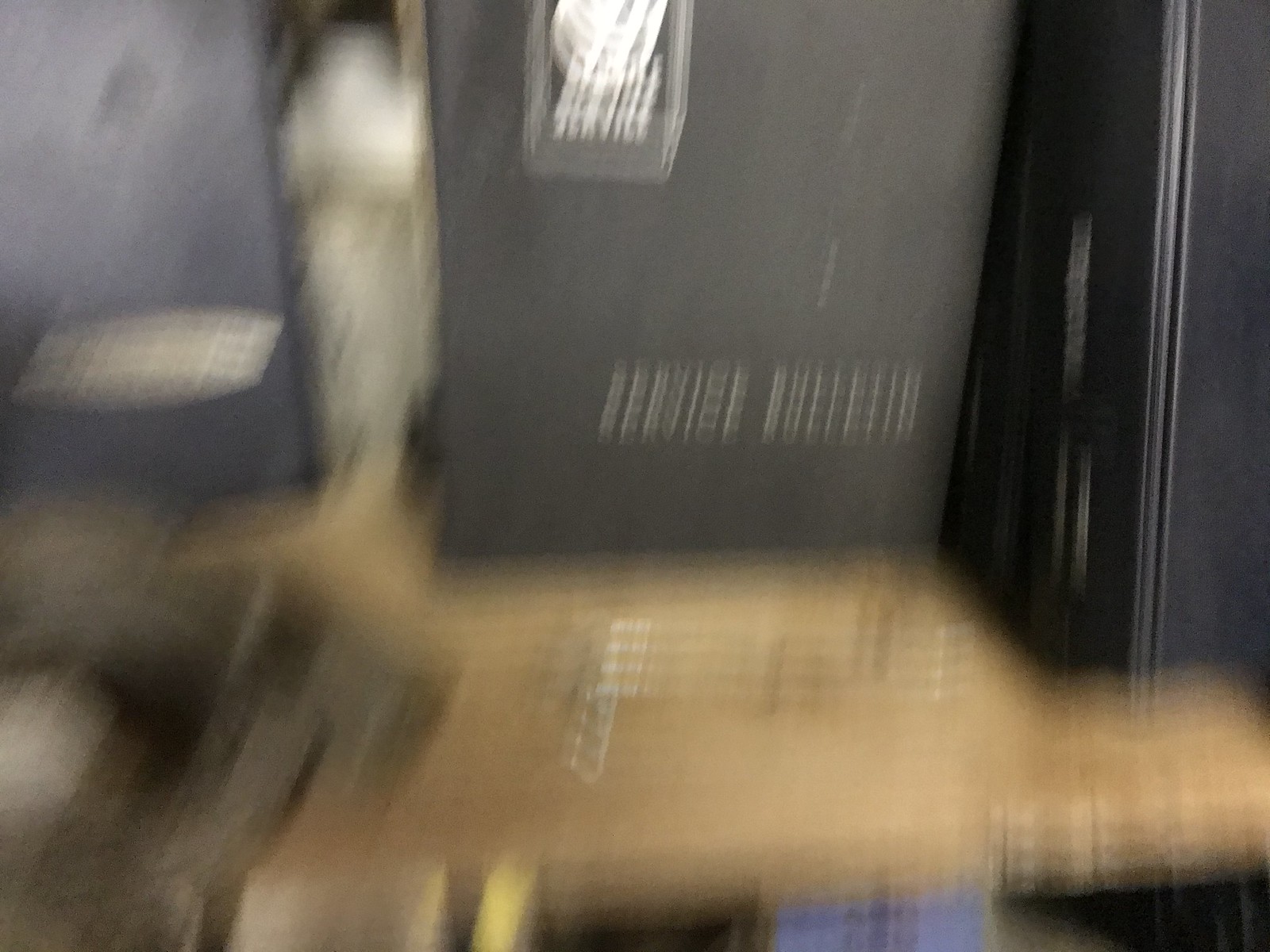The photograph is notably blurry, depicting three black rectangular objects positioned on a tan or light brown surface, which appears to be a wooden platform or table. The central object has partially visible text that seems to read "Service Bulletin." The setting features grey metal fixtures emerging from grey walls, adding to the scene's industrial or utilitarian feel. There is also a navy blue object towards the left and additional silver elements within the composition. While the image lacks clarity, the arrangement suggests a deliberately staged setup, with a possible context leaning towards an official or mechanical environment.